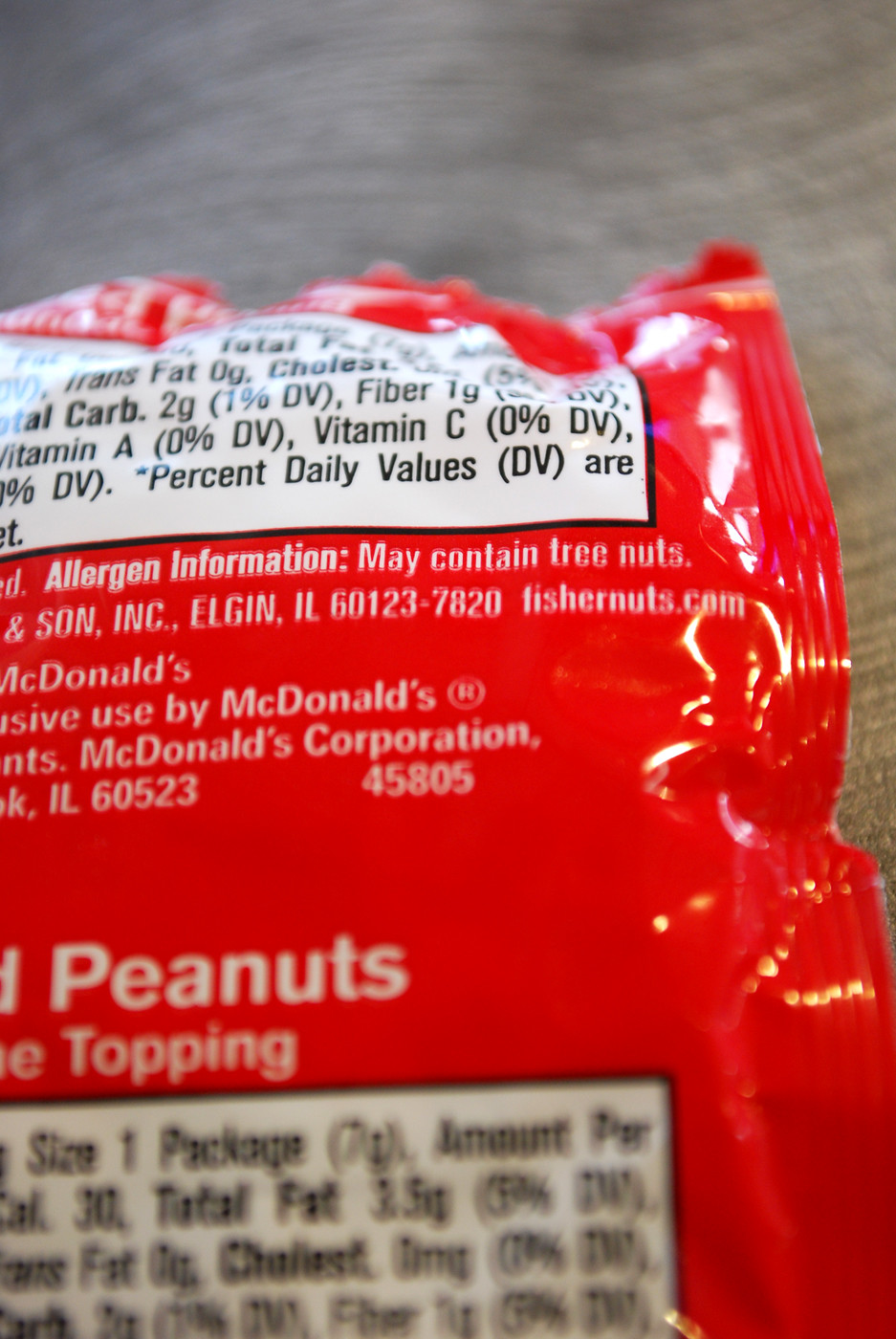A detailed caption for the image you described could be:

"A red package of peanuts, partially visible due to the top being cut off. The label prominently displays the word 'Peanuts' at the bottom with images of peanuts underneath. The nutritional information is listed on the front of the package, including details such as carbohydrates, fiber, and Vitamin C percentages of daily value. There is also allergen information indicating the product contains tree nuts, with additional text referring to 'Sun Inc.' and a series of numbers: 601237820. The packaging features the McDonald’s Corporation branding. The photo captures an indoor setting with the light from a yellow indoor source on the right and natural outdoor light from a window. The background suggests a non-wooden, likely smooth surface."